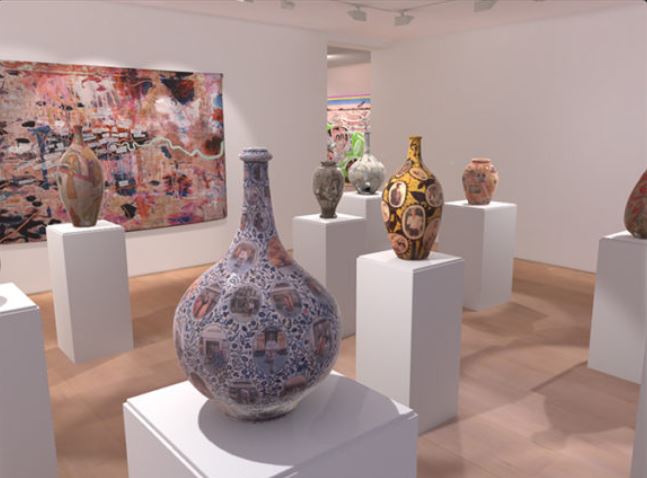The photograph depicts an art gallery with white walls and a light beige floor. The floor is arranged with tall, white columns diagonally across the space from the bottom left corner to the top right. Each column supports a ceramic vase of various shapes and colors, including blue, yellow, gray, silver, cream, orange, pink, green, brown, lilac, and shades of wine. In the foreground stands a blue vase. Behind it to the right is a yellow vase, and diagonally behind that one to the left is a gray vase. Further back, there is a silver vase, with a cream-colored vase to its right and another cream-colored vase to the left of the blue vase in the foreground. On the left wall hangs a large rectangular abstract painting in many colors without a clear image, prominently featuring browns and wines with touches of blue and black. Another similarly abstract painting is visible in the background on the right side, partially covered by walls. Ceiling lights spotlight both the paintings and the vases, enhancing the display.